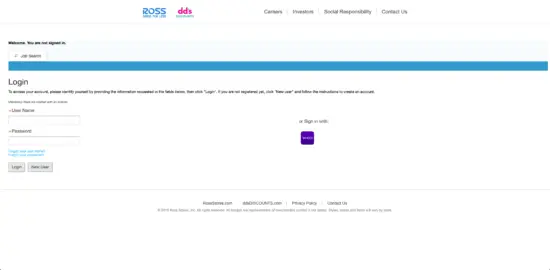The image likely depicts a login interface, potentially an admin panel for Ross Dress for Less. The Ross Dress for Less logo appears at the top, accompanied by a DDS logo in pink to its right, whose purpose is unclear. The image shows a menu that is difficult to read but includes options such as "Careers," an unreadable option, "Social Responsibility," and "Contact Us."

Below the menu, a welcome message indicates that the user is not signed in. A blue line runs horizontally across the width of the screenshot with the word "Login" beneath it. There is a lengthy line of text in an exceptionally small font below the login header, making it unreadable. Two input fields are present for entering a username and password. Additionally, there are blue disclaimer texts or possibly links to terms and conditions.

The interface includes a login button and an option for new users to register. At the bottom of the center area, an unreadable footer is present. Another option says "Or sign in with," followed by a square icon or logo that appears to be purple. The screenshot is notably small, rendering many of its details difficult to discern.